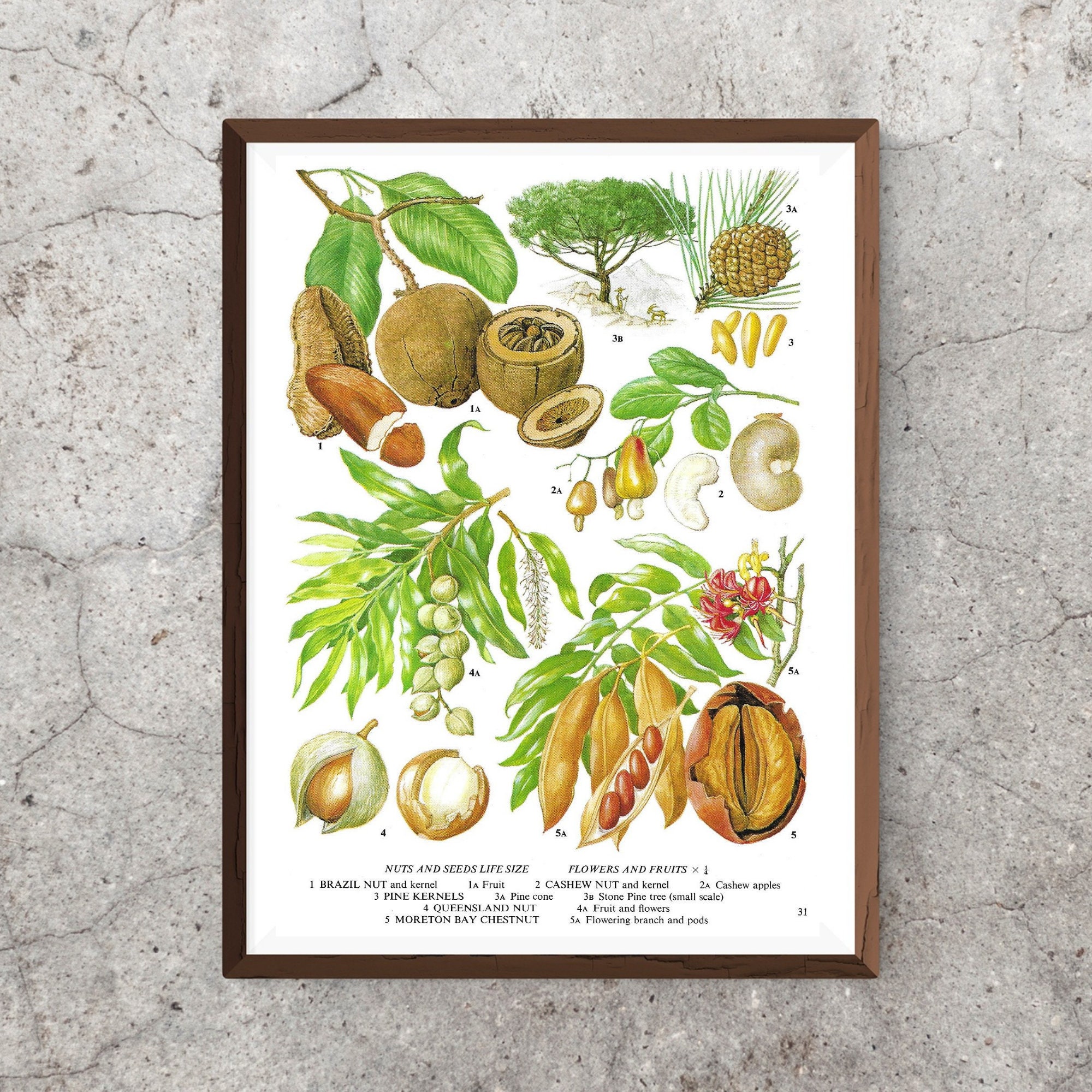The image is an illustration of various plants, specifically nuts, seeds, flowers, and fruits, presented in a detailed botanical print. It is framed in a dark wooden frame, which shows some cracks, and is placed against a dark gray, cracked stone wall. The vibrant and bright illustrations in shades of brown, green, and yellow stand out against the white background.

At the bottom of the print, there is a descriptive key in black text. On the left, it reads "Nuts and Seeds, Life Size," and on the right, "Flowers and Fruits x 1." Each labeled illustration is numbered and in some cases, includes a letter to denote different parts of the plant:

1. **Brazil Nut and Kernel** - Positioned in the top upper left-hand corner, with "1A" indicating the fruit.
2. **Cashew Nut and Kernel** - Located towards the middle right-hand side, labeled "2A" for Cashew Apples.
3. **Pine Kernels** - Illustrated in the top upper left-hand side along with "3A" the Pine Cone, and "3B" the Stone Pine Tree at a small scale.
4. **Queensland Nut** - Shown in the middle left-hand side, with "4A" denoting the fruit and flowers.
5. **Morton Bay Chestnut** - Positioned on the bottom right-hand side, with "5A" for the flowering branch and pods.

These detailed descriptions explain the growth and appearance of each nut and seed, both in their shells and without, providing a comprehensive visual guide to these plant species.